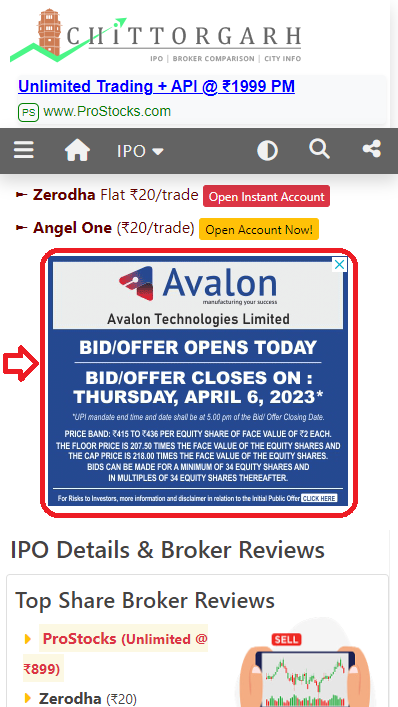**Captivating Image Description:**

At the top of the image, the name "CIITTOGARH" is prominently displayed, suggesting it is a brokerage company. Accompanying the name is a green trade line, resembling the bar graph commonly seen in stock trading platforms. Below, text reads "IPO Broker Comparison City Info," followed by a blue hyperlink stating "Unlimited Trading Plus API at 1999 PM."

Further down, in green text, the link "PSWWW ProStocks.com" is seen. Below this is a gray banner featuring several icons: three horizontal menu lines, a home icon, an IPO dropdown triangle, a circle that is half white and half black, a search icon, and a share icon.

The image then lists names of other companies, such as "Zero.Flat" with a prompt to "Open Instant Account," and "Asia One" advertising "$20 Trade" with an "Open Account Now" call to action. 

Central to the image is a square outlined in red followed by blue, containing the text "Avalon, Avalon Technologies Limited." It informs viewers that the bid offer opens today and closes on Thursday, April 6th. Beneath this, the text "IPO Details and Broker Reviews" affirms the site's trading focus.